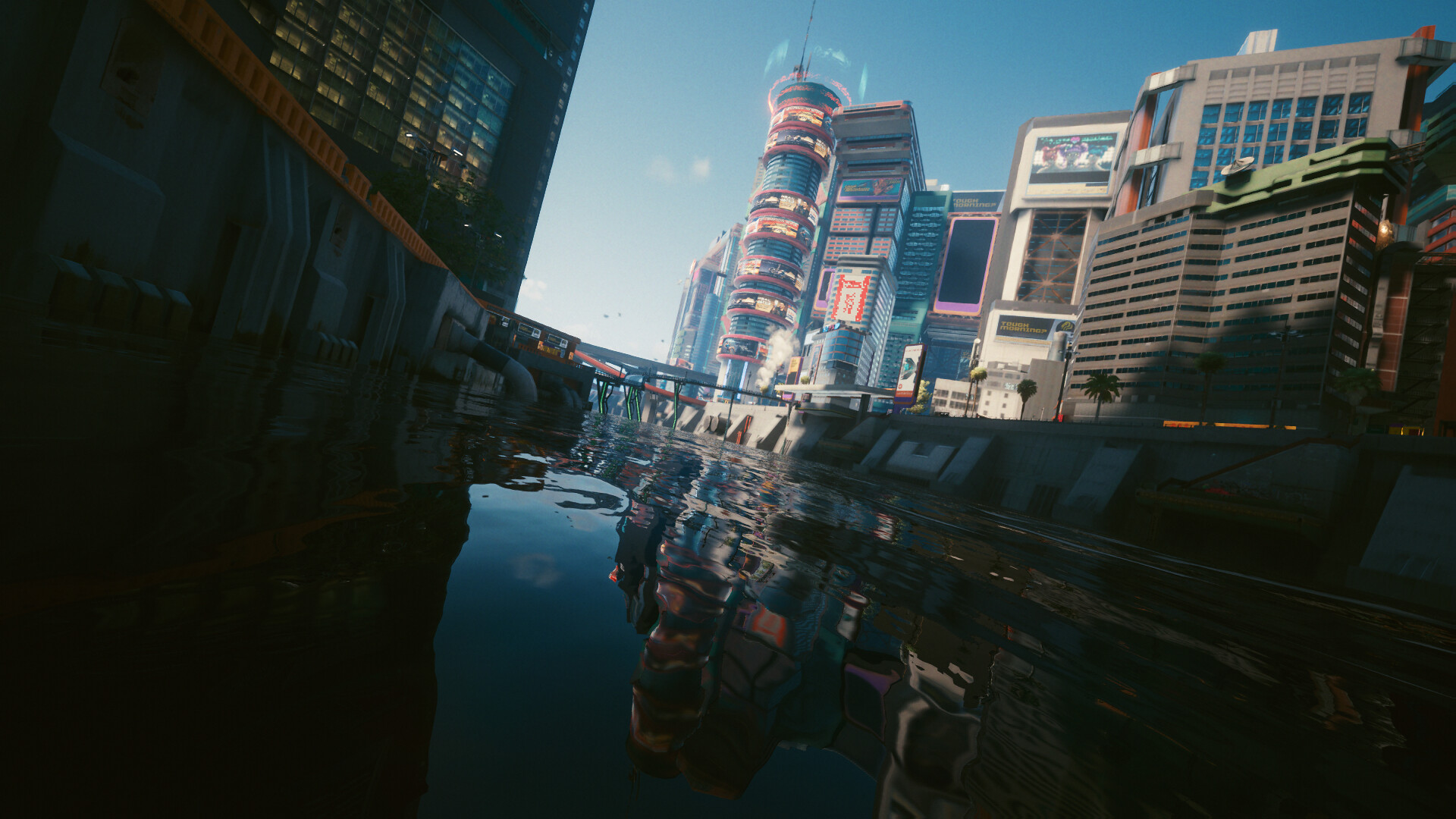This illustration depicts a vibrant, futuristic cityscape centered around a large man-made canal. The waterway, situated prominently in the foreground, reflects the towering structures that line its banks, enhancing the scene's dynamic feel. On the right side of the image, an array of buildings forms a striking skyline. Notably, there's a shorter brown building with black lines, a taller one adorned with numerous windows, and another featuring a prominent billboard. Additionally, cylindrical towers, covered in circular digital billboards, rise majestically, some topped with swirling holograms. The architecture blends ultra-modern elements with traditional designs, showcasing colorful facades in hues of teal, red, and yellow, conjuring an almost Lego-like appearance. Meanwhile, the left side of the illustration reveals portions of a massive building with numerous windows, adding balance to the composition. In the background, a blue sky provides a serene backdrop, contrasting with the city's bustling energy. The overall effect is a compelling vision of a futuristic urban landscape, meticulously detailed and rich in contrasting architectural styles.